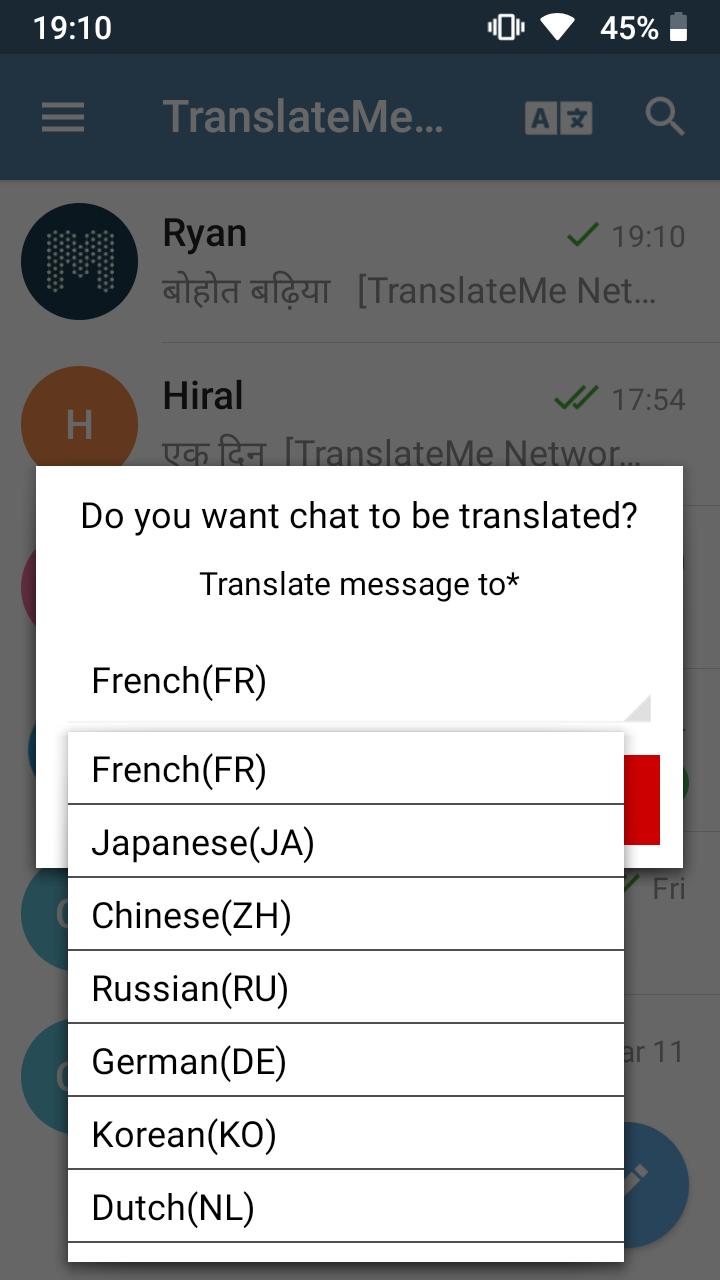The screen features a grayed-out background with two active pop-up windows overlaying it. In the background, the time "19:10" is visible along with signal strength indicators consisting of two lines increasing in size to the right, followed by a white-outlined rectangle, and two lines decreasing in size. A fully white fan icon shows a charge of 45% with the lower half of a battery symbol also in white. The background screen displays three horizontal lines and the phrase "Translate Me." Below that, there is an 'A' symbol flanked by divide and times signs, a question mark, and a circle labeled "Ryan," accompanied by text in what appears to be Sanskrit. Additionally, there is an 'H' within an orange circle labeled "Hyrule," again followed by text in Sanskrit. 

The foremost pop-up is a white window asking, "Do you want the chat to be translated?" with options to "Translate to" marked by an asterisk and a dropdown listing "French (FR)." 

Another pop-up window overlays this, presenting a language selection with options including French (FR), Japanese (JA), Chinese (ZH), Russian (RU), German (DE), Korean (KO), and Dutch (NL).